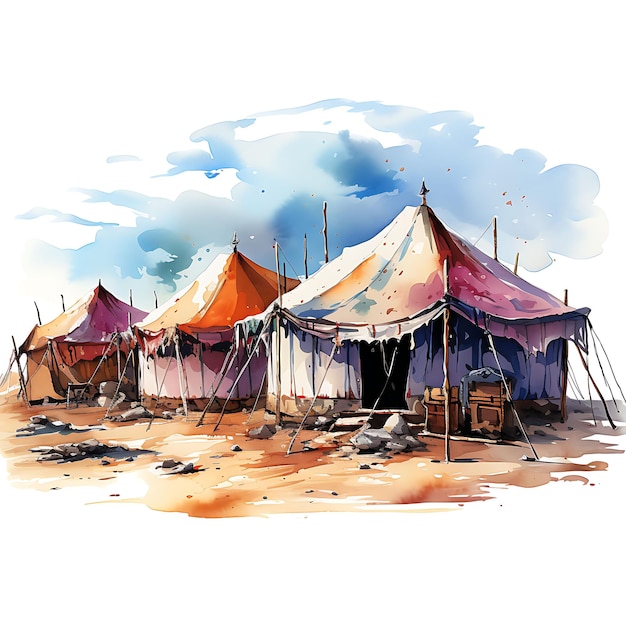This image, set against a solid white background, depicts a picturesque arrangement of three tattered tents, reminiscent of those at a vintage carnival, on a sandy or dirt ground that features both light and dark brown patches interspersed with some white areas and small rocks. The tents showcase a whimsical array of colors with worn and weathered appearances. 

The tent in the foreground at the center stands out with a base of white, mixed with hues of brown, purple, blue, and orange on top. Moving to the left and slightly further back, the second tent displays a predominantly orange and white top with a body of light pink or white, accentuated with gold and beige. The tent furthest to the left, situated even further back, features a brown and purple top with dominant brown hues on its body, infused with a touch of red and tan. The poles supporting these tents slant diagonally, enhancing the rustic charm of the scene.

The rough terrain around the tents is cluttered with various small rocks and debris, including what appear to be old appliances and assorted trash, adding to the sense of disarray. Above, the sky is dominated by an overcast ambiance, rendered in shades of white and gray, with some areas depicting blue clouds, suggesting a cloudy day. This intricate watercolor painting captures the nostalgic essence of a bygone carnival, amidst a landscape of decay and color.